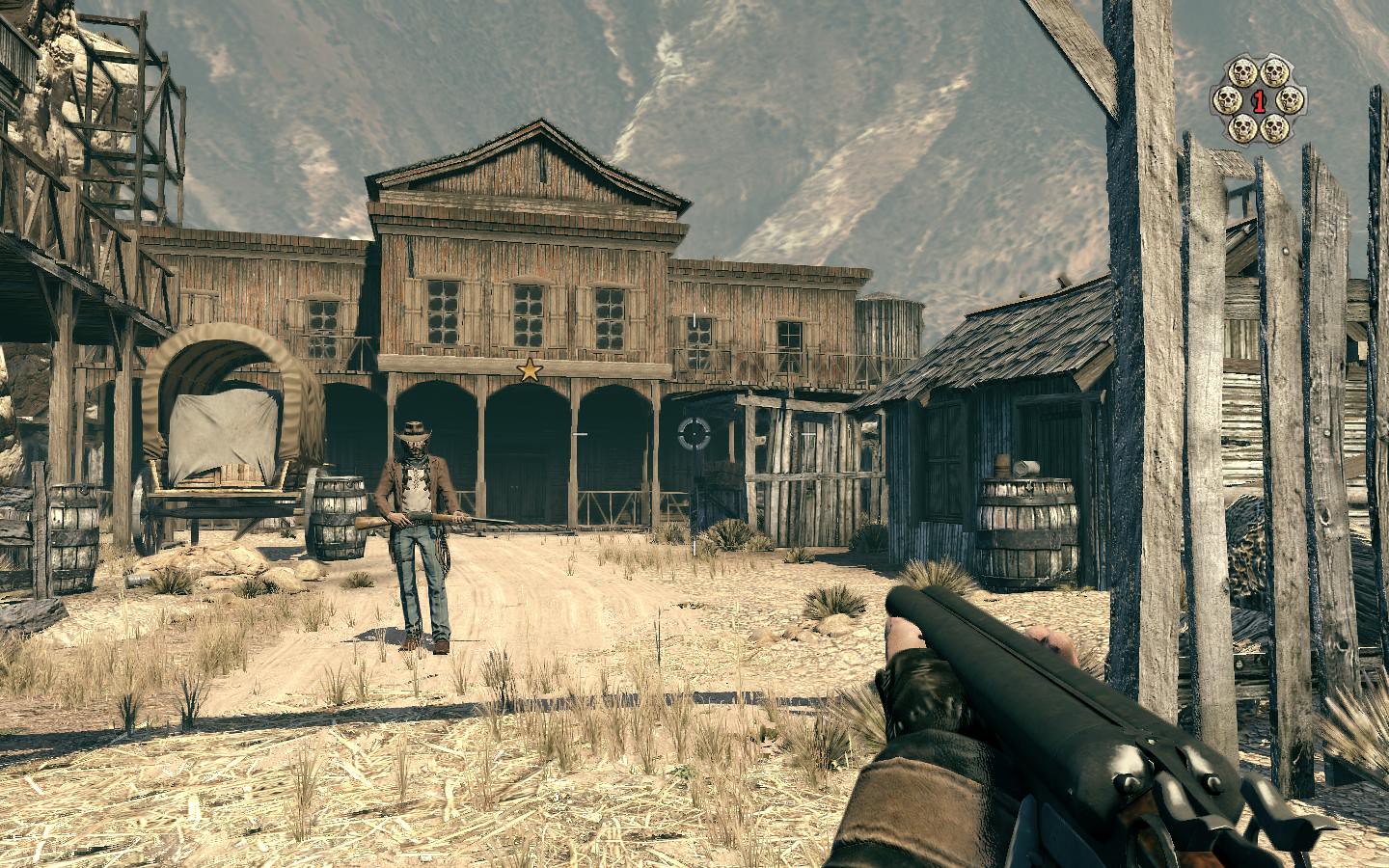The image is a detailed, animated depiction of a Western town, likely from a video game reminiscent of the Red Dead Redemption series. In the foreground, the perspective suggests a first-person view, with a character aiming a double-barrel shotgun, their hands clad in fingerless leather gloves and a light brown cuff. The scene centers around an old, brown wooden building that bears a prominent sheriff's star above a central arch doorway, flanked by two additional arches. A sheriff, dressed in cowboy boots, denim jeans, a cowboy hat, and a long brown jacket, stands in front of the building holding a shotgun with a black tip. To the left of the sheriff, a covered wagon with large wheels is visible, adding an authentic touch to the deserted, tumbleweed-strewn street. In the backdrop, a steep, imposing mountain rises, its peak out of view, giving the impression of a setting that could be in Colorado or Utah. A small shed with a grayish wood barrel in front stands to the right, completing the rustic Western town atmosphere.